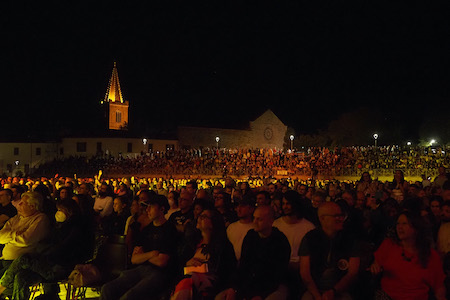In this nighttime image, a very large crowd is gathered outdoors in front of an imposing, old stone building that resembles a church, complete with a tall, illuminated steeple. The building features a prominent round window at the front and several square windows along its sides. The scene is lit predominantly by numerous yellowish lights that cast a warm glow over the entire area, creating a striking contrast against the perfectly black night sky. The crowd, which appears to be seated in rows possibly arranged on bleacher-style seating that angles upwards, is densely packed and all facing towards a presumed focal point in the distance. The demographic of the crowd seems to be mostly older individuals, suggestive of a religious or ceremonial event rather than a youthful gathering. The atmosphere is charged with anticipation as the multitude of people gaze intently ahead, possibly watching a performance or a significant presentation.